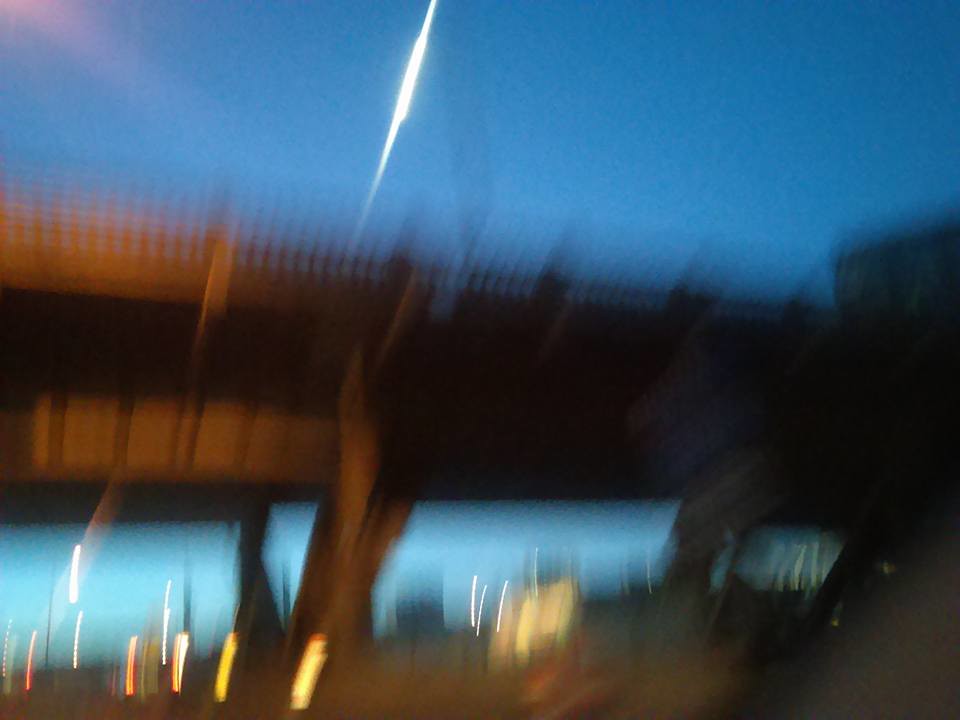A blurred image captures a brown bridge suspended over a body of water, with light blue water blending seamlessly into the similarly colored sky. Unusual light effects appear as dashes at the bottom and a prominent light beam descends from the top, accompanied by a pinkish ray originating from the left corner. The bridge is supported by what seem to be metal legs, lifting it off the ground. It features a metal-like railing with a horizontal design.